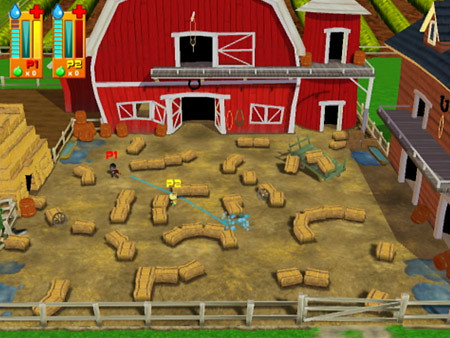The image is a vibrant, cartoon-esque screenshot taken from a video game. At the top, there are indicators for Player One and Player Two, each with graphical meters and icons. Player One’s water meter is down by two bars, while their health is fully replenished, signified by a full yellow bar. In contrast, Player Two has a full water meter but no yellow in their health section, suggesting they have no health left.

At the bottom of the screen, each player's status shows a green water balloon or bomb icon, with "time zero" displayed next to both players. The backdrop is a rustic farm scene, complete with a red barn resembling a classic ranch farmhouse. Surrounding the barn are hay bales and fences, adding to the agricultural ambiance.

In the scene, Player One is depicted in red and is actively engaged, shooting a stream of water at Player Two, who is labeled in yellow. The action is marked by an animated splash of water cascading past Player Two, creating a dynamic and lively interaction between the characters.